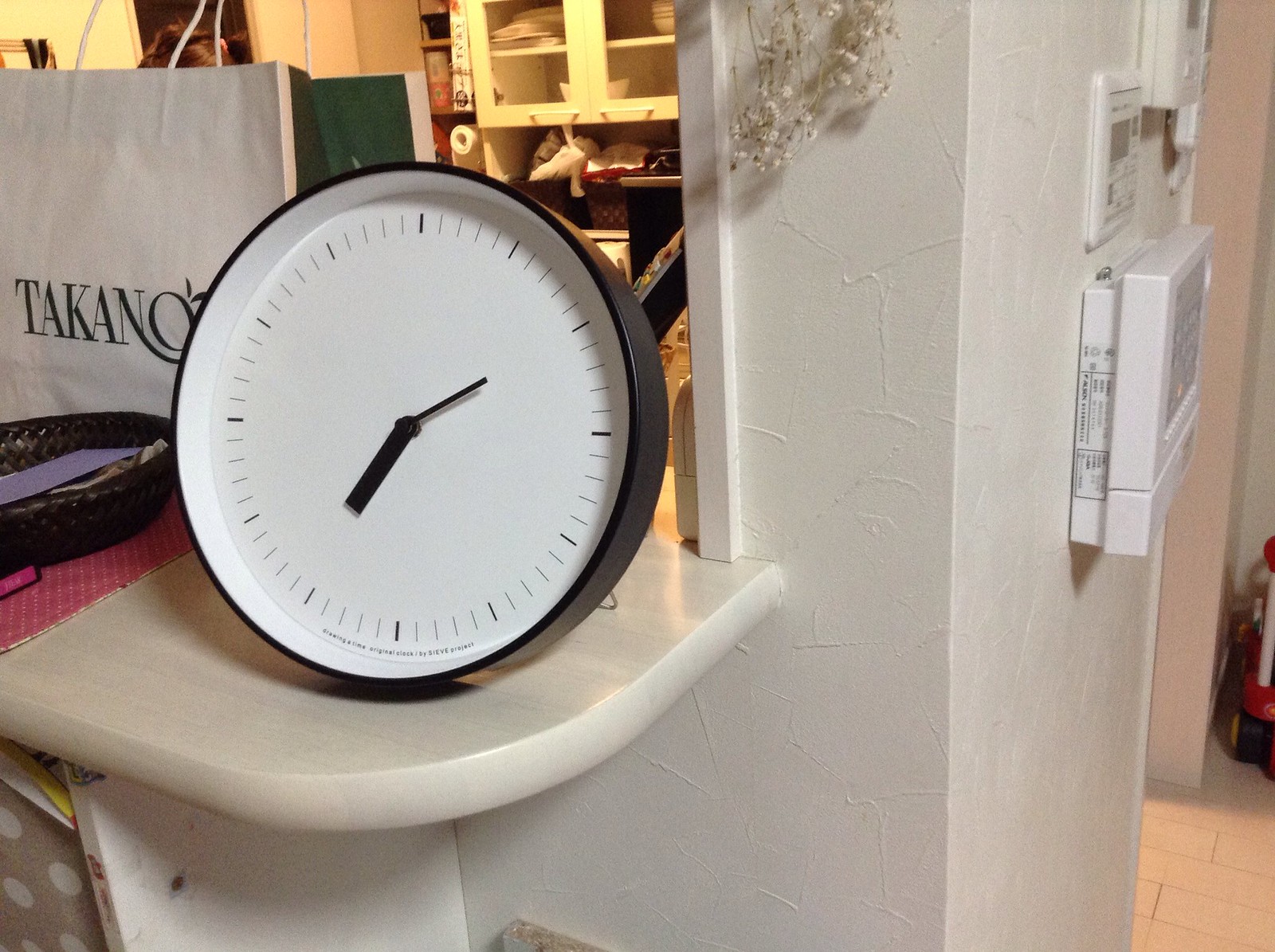In the image, there is a scene featuring a white counter, likely part of a store setup. Atop the counter sits a white T-A-K-A-N-O bag adorned with black lettering, next to a pink cloth and a brown wicker basket. The counter stands against a wall with a subtle stucco-like texture, appearing more gray due to the lighting. 

Behind the counter, an office space is visible, cluttered with shelves and various items. To the right of the counter, a black-rimmed, circular clock is mounted on the wall. The clock's face is modern in design, featuring a clean, white surface without numbers. Dark black lines mark the hours at positions equivalent to 12, 5, and 10, with thinner gray lines denoting the minutes in between.

Directly beneath the clock is a thermostat, and a larger unidentified unit is positioned even lower on the wall, partially obscured in the image. The clock shows the time as approximately 2:37, indicated by a thicker minute hand and a slightly thinner, similarly sized hour hand.